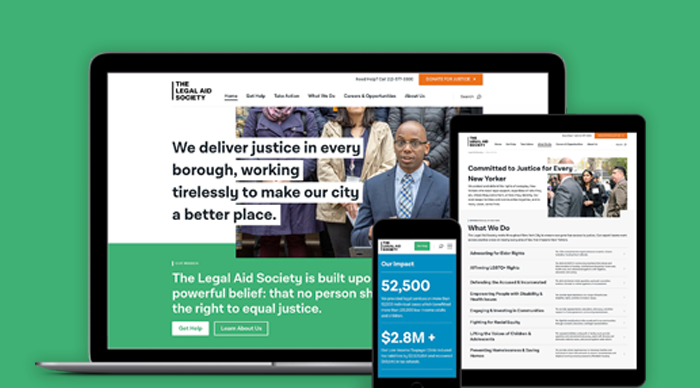The image showcases a series of digital devices in front of a vibrant green screen background, likely intended for chroma key editing. Centrally, a laptop displays an advertisement for the Legal Aid Society, featuring the tagline: "We deliver justice in every borough, working tirelessly to make our city a better place." The laptop screen also includes an image of a man in a suit giving a speech, accompanied by several individuals in jackets standing behind him. Text beneath the image reads, "The Legal Aid Society is built upon the powerful belief that no person should be denied the right to equal justice." Additionally, the screen features actionable buttons labeled "Get Help" and "Learn More About Us."

Overlaying the laptop, a tablet screen highlights the message "Committed to justice for every New Yorker," possibly accompanied by another picture of the same group of people. Below this message, a heading states "What We Do," hinting at further details about the organization's activities.

In front of both the laptop and the tablet, a phone screen is visible with the heading "Our Impact." It prominently displays the figures $52,500 and $2.8 million+, indicating significant metrics relevant to the Legal Aid Society, though the accompanying descriptions are not fully legible. The ensemble of devices and information suggests a multifaceted advertisement promoting the mission and impact of the Legal Aid Society.